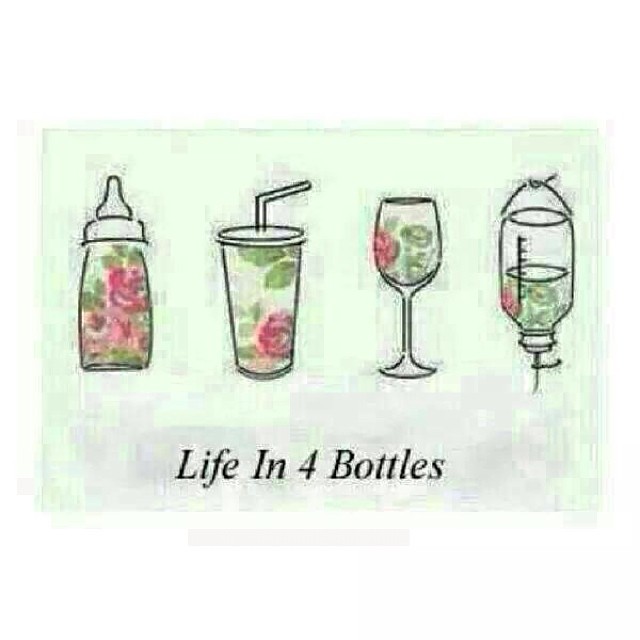The image is a pixelated, low-quality drawing titled "Life in Four Bottles," showing four stages of life through different containers, each filled with a floral pattern of green leaves and red or pinkish flowers. The first bottle is a baby bottle with brown and gray coloring, followed by a fast food soda cup with a lid and straw. The third container is an empty wine glass, and the fourth is a hanging IV drip bag, also with brown and gray liquid. The background is an off-white, very light mint green and white, with a grainy and pixelated texture. At the bottom of the image, the title is printed in black font, using the number four to denote "Four."